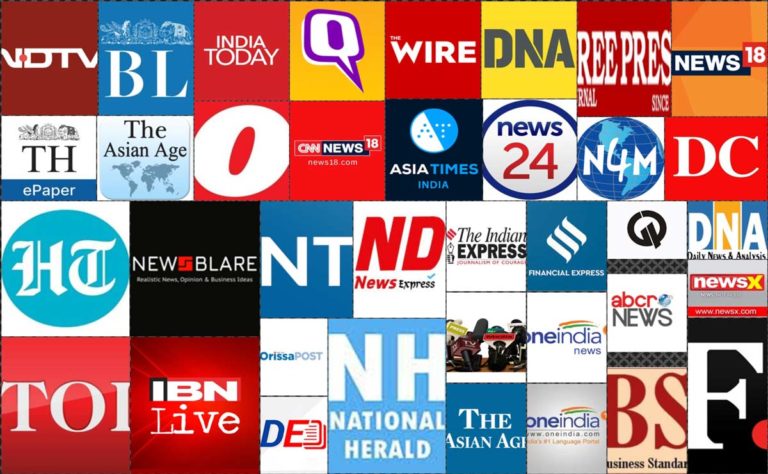This image is an intricate animated collage showcasing a variety of media logos and symbols. Dominating the left side is "NDTV" written in white font against a red background. Adjacent to it is "BL" followed by "India Today". Below, there is a picture depicting a queue. Other prominent logos include "The Wire", "DNA" (Daily News and Analysis), "Repress", "News 18", and "The Paper". "The Asian Age" logo is also notable, featuring an image of a map. A striking red square with a large "O" in it stands out among the others. Additional logos displayed are "CNN News 18", "Asia Times India", "News 24", and "CNN 4M", which includes an image of a globe. "DC", "New Blair", "NT", "The Indian Express", and "IBN Live" also make appearances. Lastly, the collage includes "NH National Heritage", "ABCR News", "India", and "Business Standard". The collection of logos against a vibrant animated background serves as a testament to the diversity and multitude of media outlets present in the industry.